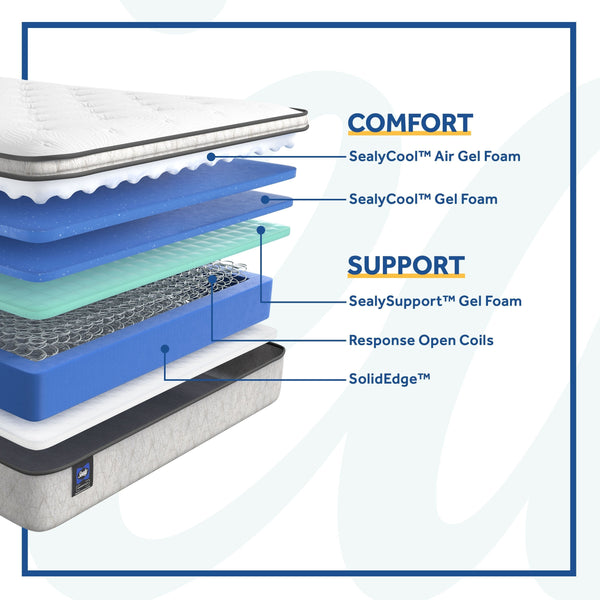This advertisement for a Sealy mattress features a square-shaped graphic with a clean white background and a blue border. Dominating the right side of the image is a detailed diagram of the mattress showcasing its various components through layered cross-sections. The topmost layer of the mattress is richly blue, transitioning to gray at the bottom, with interior layers in shades of blue and green. These layers are meticulously labeled with corresponding text and lines that identify their function and material.

From top to bottom, the layers are designated for different aspects of comfort and support: "Comfort" boasts the Sealy Cool Air Gel Foam and Sealy Cool Gel Foam, highlighted with an underlined yellow line. "Support" features the Sealy Support Gel Foam, also underlined in yellow. The "Response" layer includes open coils made of stainless steel, and the "Solid Edge." Each layer’s contribution to the overall support and comfort of the mattress is emphasized, suggesting a superior level of relaxation and stability. The left side of the image shows only the right corner of the mattress, enhancing the focus on the cross-sectional details. This ad illustrates the well-engineered layers that promise a comfortable sleeping experience.